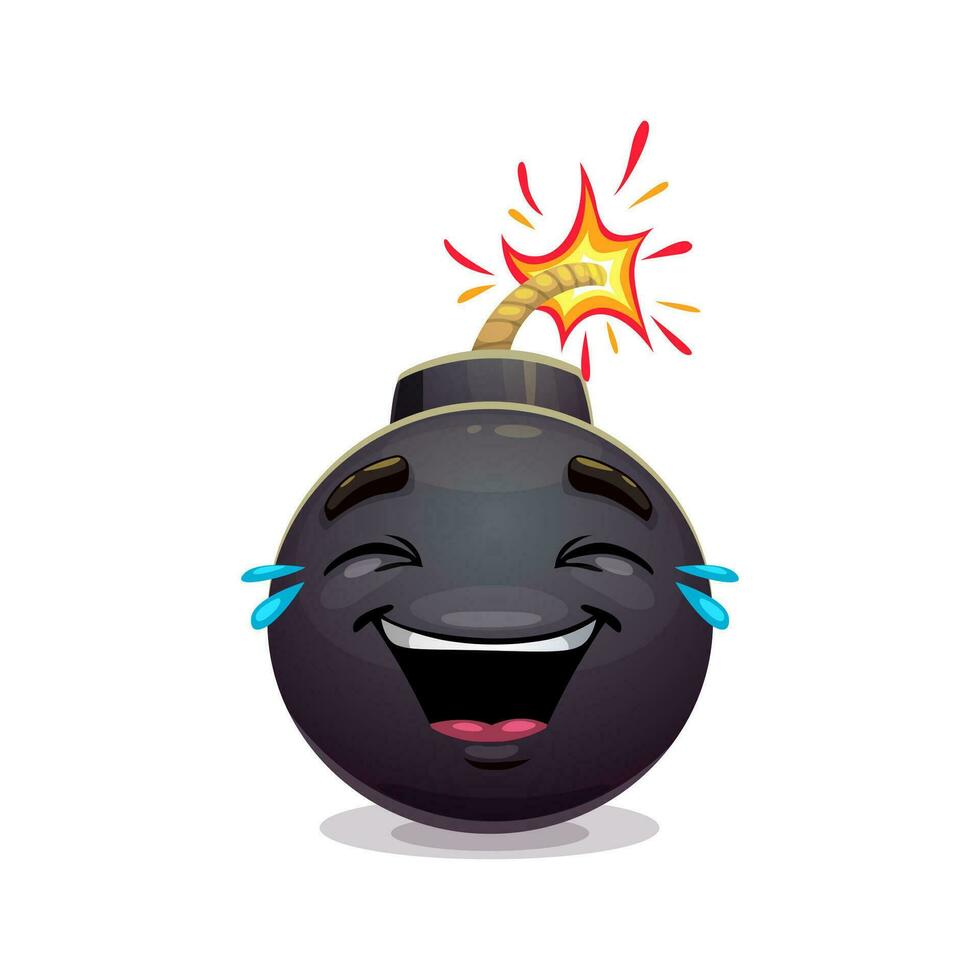This image is a clipart-style depiction of a black bomb with a highly expressive anthropomorphic face. The bomb features thick black eyebrows and eyes that are squinted shut in laughter, with blue teardrops streaming from each eye to emphasize its heavy laughter. The wide-open mouth reveals white teeth and a pink tongue, contributing to its animated, jovial expression. The bomb is topped with a rope fuse that is actively burning, illustrated by yellow, orange, and red flames, signaling that it's been lit. This hand-drawn or cartoon-like bomb rests on a completely white background, with a subtle shadow beneath it, reinforcing its buoyant, upright posture.